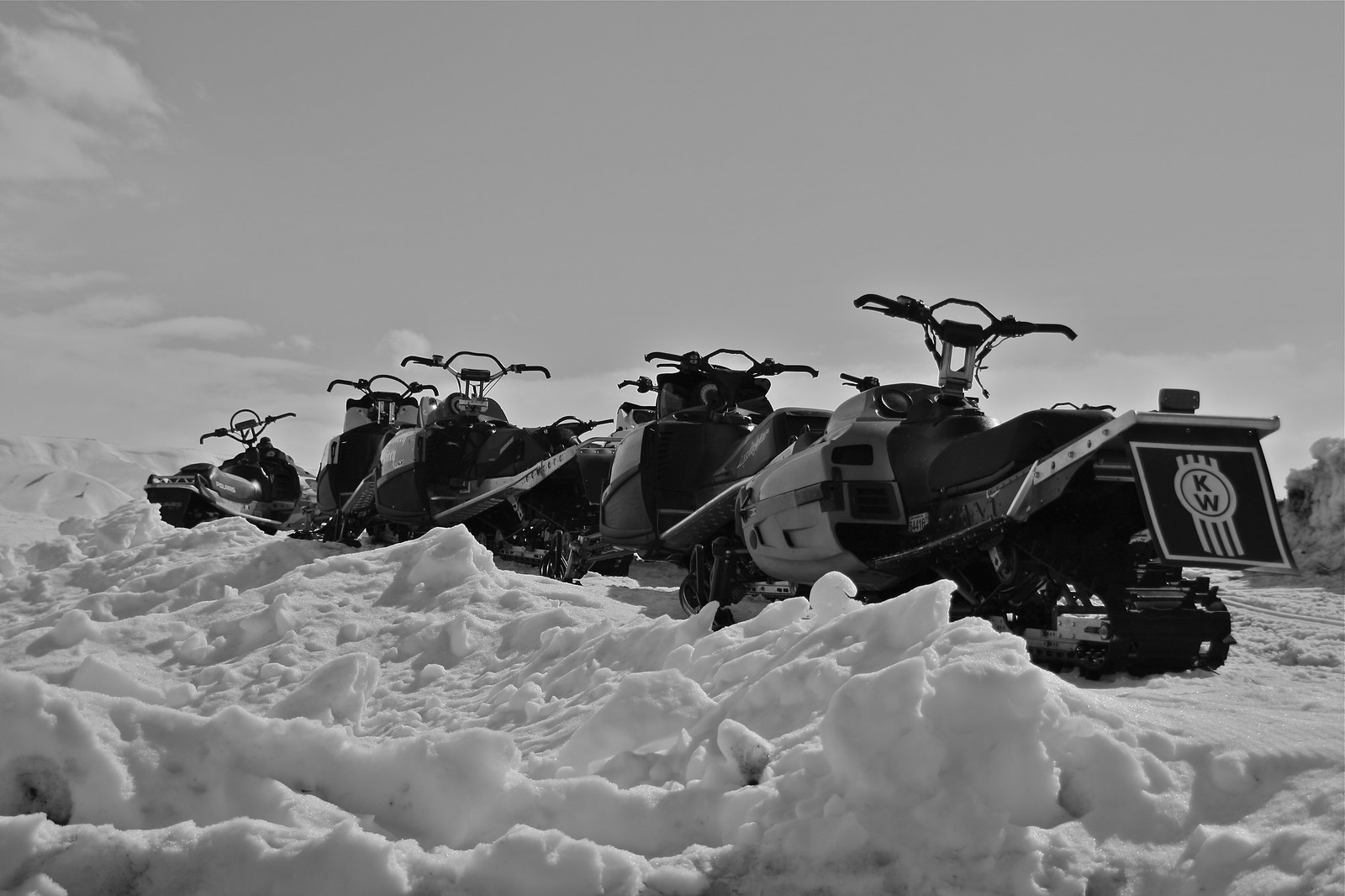The black and white photograph captures an outdoor scene viewed from a low angle, making it seem as though we are lying down and looking slightly upward. The setting reveals a clear sky with a few scattered clouds positioned in the top left and bottom middle of the image. The ground is covered in snow, which appears chunky and ice-like in some parts, particularly toward the left side leading up to a hill-like structure. In the middle of the composition, five snowmobiles are lined up in a straight row, each seemingly built for one or two riders. Notably, the last snowmobile in the line displays a flap on its back featuring a design—a "KW" within a white circle with vertical lines behind it. The black and white color scheme of the photo adds an element of curiosity, leaving one to wonder about the specific event and the reasoning behind the monochromatic choice.